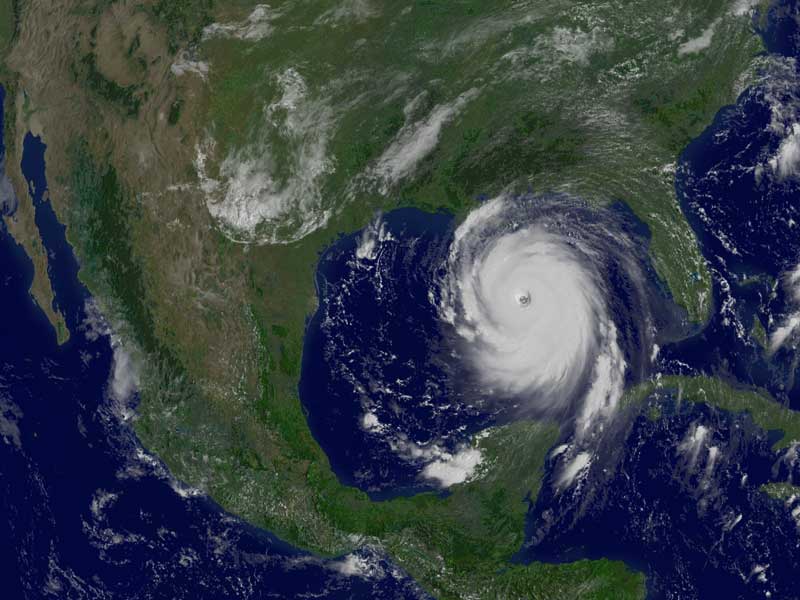This overhead, space-view image depicts the United States and Mexico with a significant focus on the Gulf of Mexico. The landmasses of the United States and Mexico are colored in shades of green and brown, while the surrounding waters are a deep navy blue. Dominating the center of the Gulf of Mexico, a white, swirling hurricane is distinctly visible, illustrating a powerful storm system initiating with a circular wind movement pattern. This formation is surrounded by scattered clouds on either side. Above the Gulf, thin, wispy clouds stretch across the U.S., while more substantial cloud cover is observable in the top right and bottom left corners above the water. Additionally, the Mexican coastline to the left is lined with clouds, highlighting adverse weather conditions. This detailed image conveys the impending severity of the hurricane and its potential impact on the Gulf Coast and adjacent regions.